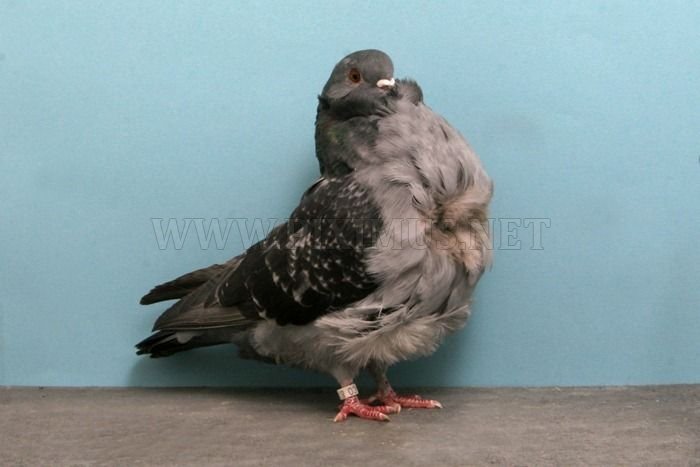In this image, a fluffy bird stands at the center on a concrete floor with a slight brownish tint. The wall behind it is painted a pretty robin's egg blue. The bird, appearing somewhat overweight, is a mix of shades with a light, tannish chest and a darker gray-brown back and head. Its feet are a dark pink, each adorned with talons and a wooden tag that seems to have a number, possibly "03," though it’s hard to discern. Additionally, the image features a very faint watermark, outlined in white and blending into the scene, which seems to read "www.heximus.net." The environment suggests an indoor setting, possibly a specialized room or a basement, designed for housing such birds.